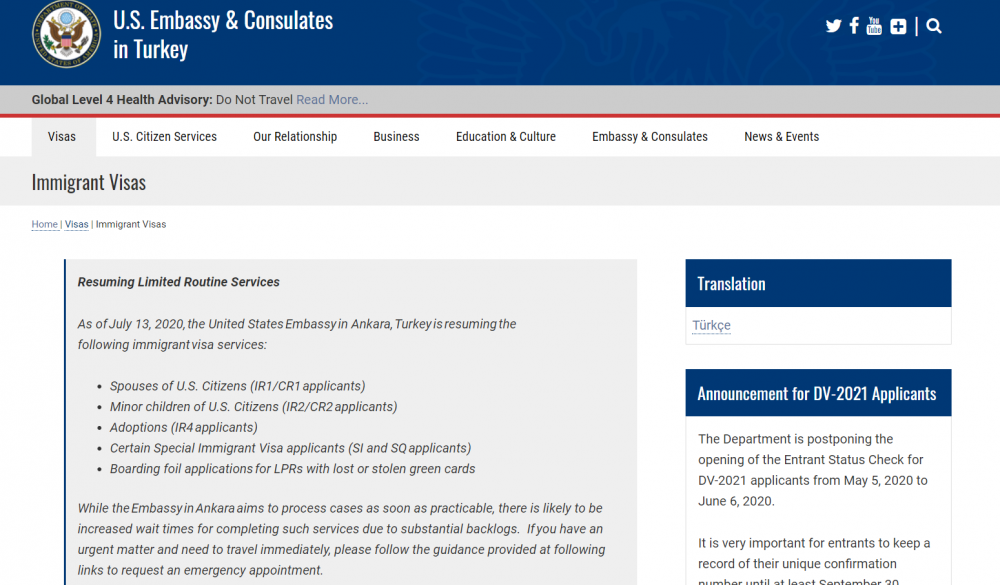In this image, the top portion prominently features a blue banner with "U.S. Embassy and Consulates in Turkey" boldly printed. Adjacent to the text, an emblem showcasing an eagle symbol, reminiscent of the U.S. Great Seal, is visible, alluding to American sovereignty. To the right of the insignia, social media icons for platforms such as Twitter, Facebook, and YouTube are displayed, offering various channels for information and communication.

Below this section, a gray bar is present with the important notice "Global Level for Health Advisory: Do Not Travel. Read More," underlining current travel advisories. Further down, several navigation sections are listed: Visa, U.S. Citizen Services, Our Relationship, Business, Education and Culture, Embassy and Consulate, and News and Events.

The Visa section is presently highlighted, revealing a detailed update on immigrant visas. Within a gray notification box, it states: "Resuming Limited Routine Services." It further specifies that as of July 13, 2020, the United States Embassy in Ankara, Turkey, resumed select immigrant visa services including applications for spouses of U.S. citizens (IR-1, CR-1), minor children of U.S. citizens (IR-2, CR-2), adoptions (IR-4), certain special immigrants (SI, SQ), and boarding foil applications for Legal Permanent Residents with lost or stolen green cards.

A note follows, indicating that while the Embassy in Ankara endeavors to expedite these processes, significant wait times are expected due to substantial backlogs. For urgent travel matters, individuals are advised to follow provided guidelines to request an emergency appointment. On the right side of the page, a translation option labeled "Türkçe" is provided for Turkish speakers.

Lastly, an announcement regarding the DV-2021 applications is displayed within another box, informing that the Department is postponing the opening of the entrance status check from May 5, 2020, to June 6, 2020.